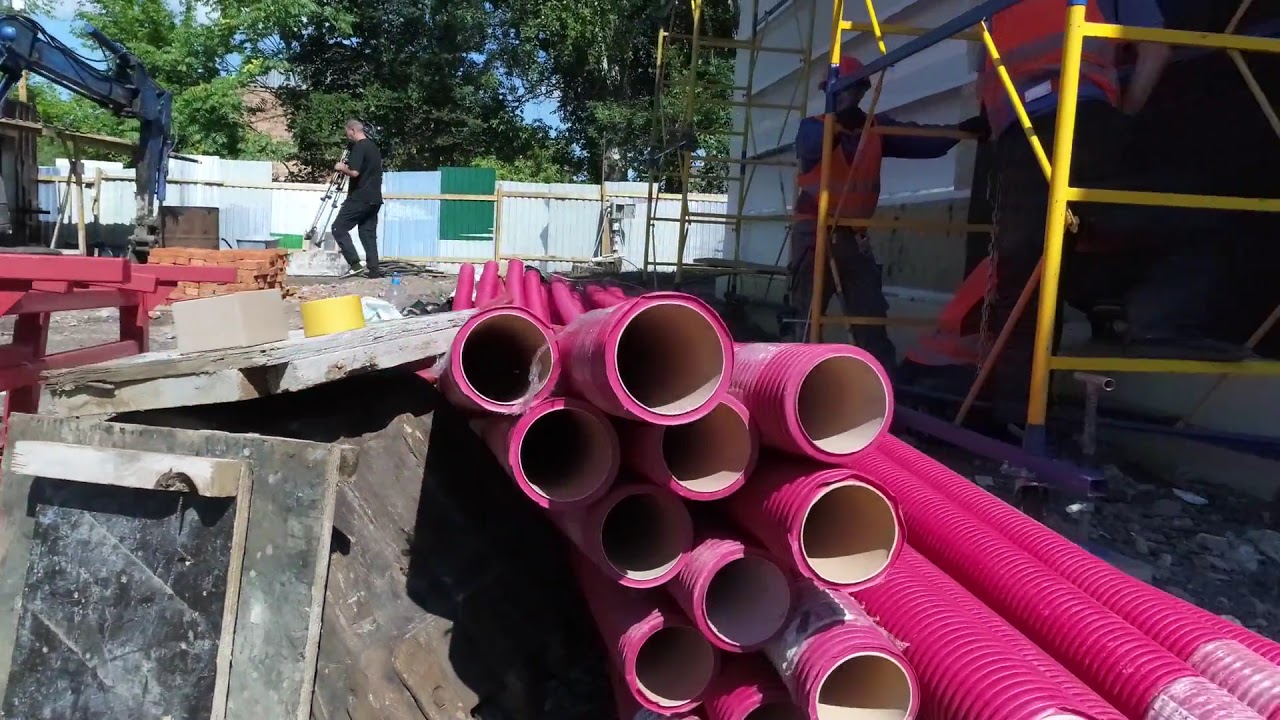The image depicts an active construction site surrounded by a backdrop of green trees and partially enclosed by a fence. The central focus is a cluster of hot pink, coiled pipes with a corrugated exterior and smooth white interior, strewn across the ground. To the right, a yellow scaffolding structure stands, beside which two men in orange hard hats, orange high-visibility vests, and jeans are working. In the distant background, another man, wearing black pants and a black shirt, is visible next to some machinery, possibly a crane, in the upper left corner. The scene is filled with various construction materials, including stacks of wood pallets and shipping containers, emphasizing the ongoing construction activity.